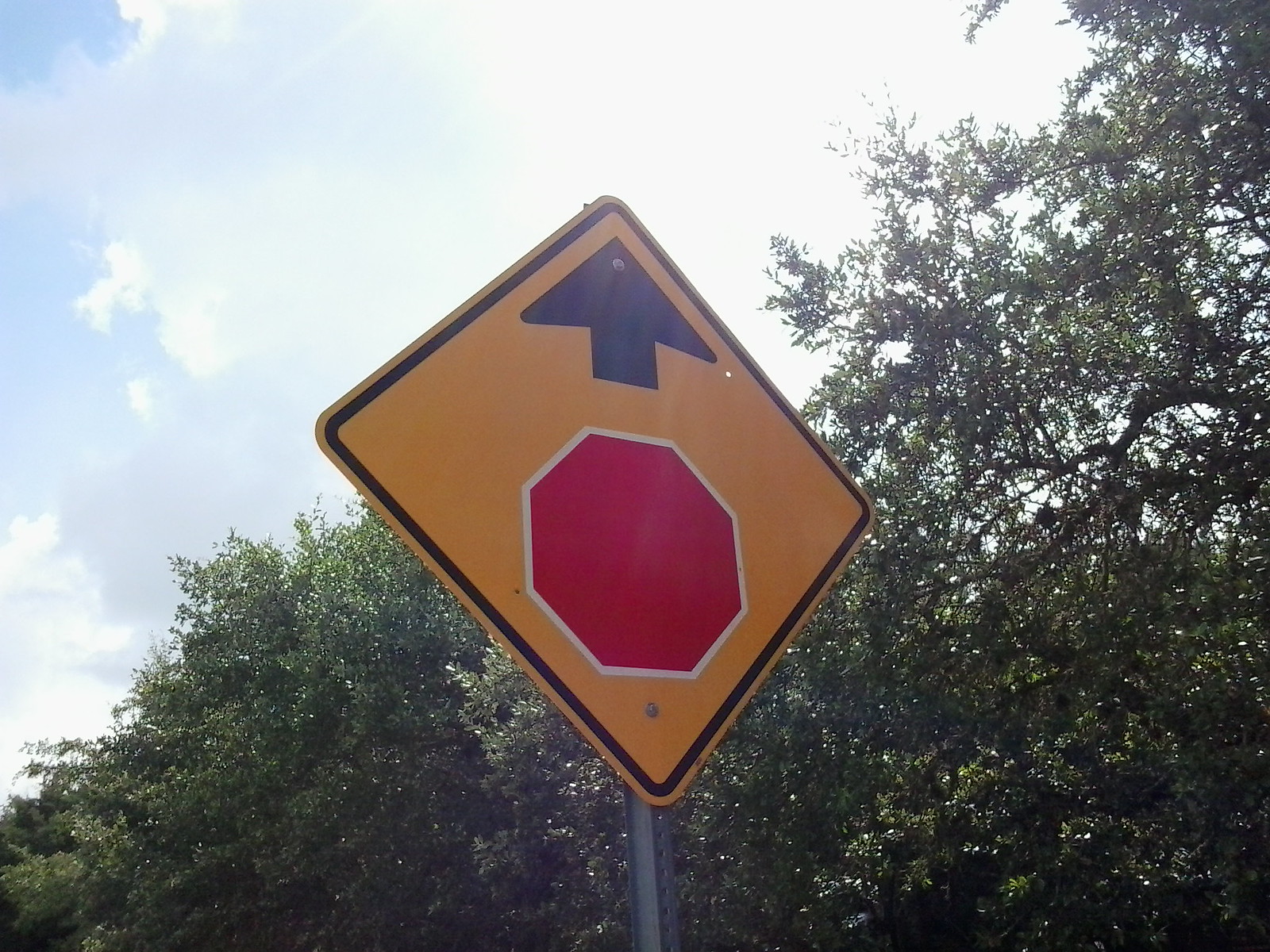In the image, a cluster of trees stands to the right under a serene sky painted in shades of light to medium blue, complemented by fluffy white clouds. Prominently featured is a yellow, diamond-shaped traffic sign outlined in black, mounted on a metal pole. The sign displays a black upward arrow, indicating a direction, and at its bottom bears the outline of a red stop sign accented with a white border. The perspective suggests the photo is taken from the street, with the photographer turning slightly to the right to capture this scene.